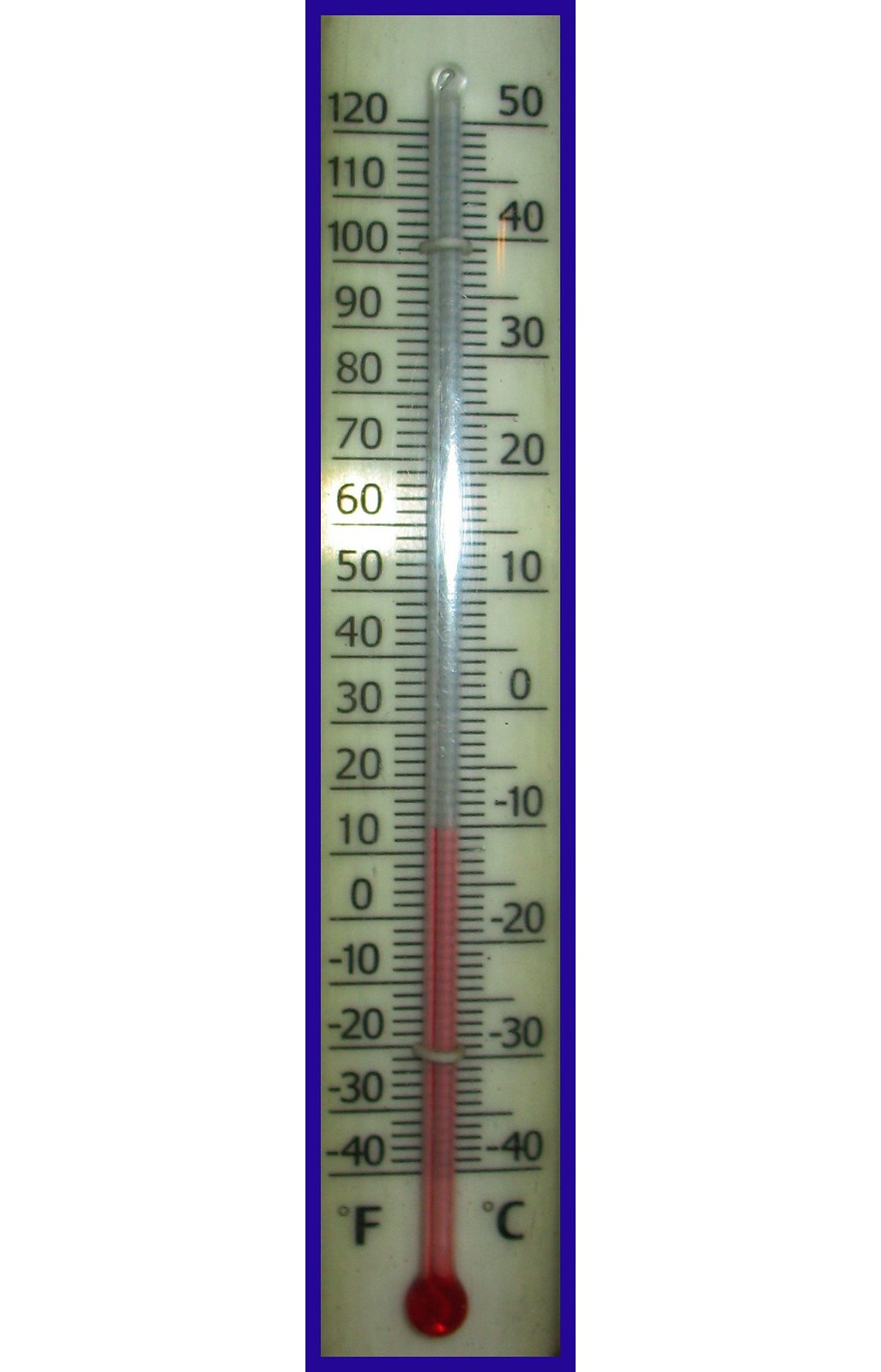This image features a detailed thermometer with a white body and blue-bordered edges. On the left side, the thermometer's scale is marked in Fahrenheit, starting from -40 at the bottom and reaching up to 120 at the top. On the right side, the scale is marked in Celsius, ranging from -40 at the bottom to 50 at the top. The temperature increments are displayed in intervals of 10 degrees, and the numbers and lines on both scales are rendered in black. 

The central portion of the thermometer comprises a clear glass tube, affixed firmly to the device. The mercury column within the tube starts turning red around -10 degrees Celsius, equivalent to approximately 12 degrees Fahrenheit, and continues in red down to the bottom of the thermometer. At the very base, there is a red circular bulb, indicating the mercury reservoir. The top and bottom of the thermometer are secured with small metal hooks, ensuring the stability of the glass tube. There are no additional notable elements within the image.